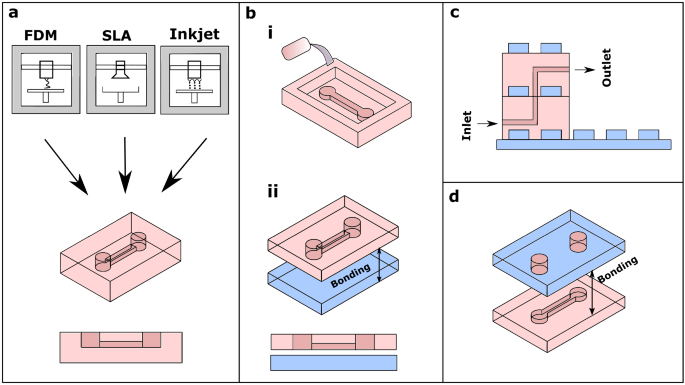The image is a detailed technical illustration of a product development process involving a printer or manufacturing system. It features a series of schematics divided into three main columns labeled A, B, C, and D, indicating step-by-step processes. The first column, labeled A, includes diagrams for FDM, SLA, and inkjet, each with arrows pointing to pink and blue components, and demonstrates initial stages of product design. The second column provides further illustrated steps, labeled as B, focusing on bonding techniques where pink components are combined with blue ones. The third column outlines the connection flow, marked with black arrows indicating inlet and outlet. The diagrams employ a plain background with text and arrows in black, while the components are highlighted in pink and blue to signify different parts and bonding processes. The steps illustrate a sequence of actions necessary for assembling or manufacturing the product, likely in an industrial or factory setting.